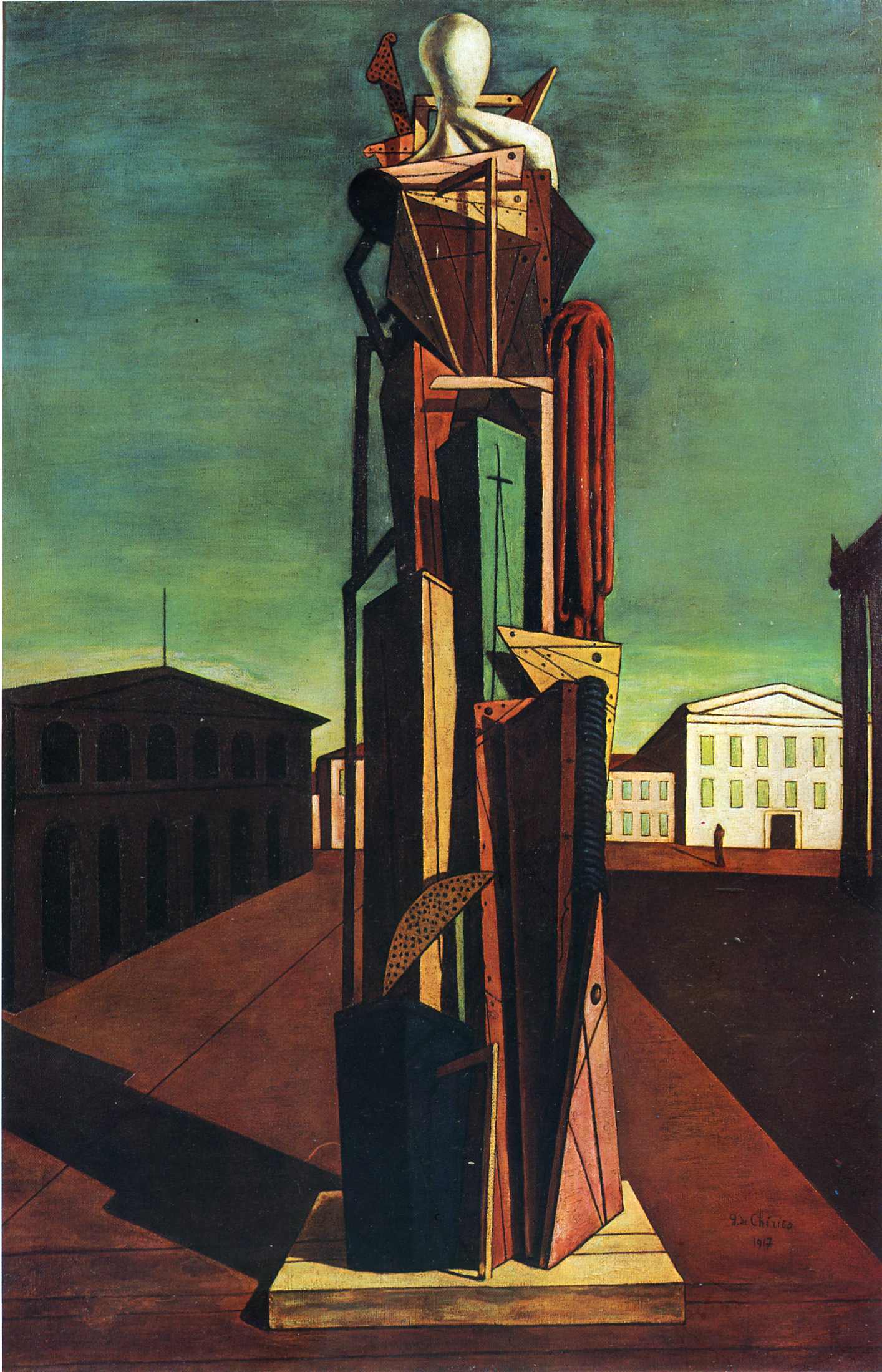This painting, abstract in nature and rectangular in shape, prominently features an eclectic sculpture placed in the center, stretching vertically from the bottom to top. This sculpture, roughly nine to ten feet tall, is assembled from diverse materials such as parts of a door, an umbrella, a box, wood scraps, tools, cloth, and a mannequin head. Its base is brown, transitioning into a mix of yellow, green, red, brown, and white elements, topped with a head-like form exhibiting a gray shadowed white hue.

The sculpture sits upon a burgundy walking path, creating a striking contrast. To the left, a shadowed building stands in the foreground, while to the right, partially obscured, other structures including what might be a church with a steeple and community or government buildings are scattered. A lone, indistinct figure appears as a silhouette near a distant building on the far right.

The lower portion of the painting is occupied by the courtyard scene, which constitutes about one-third of the image's height, while the upper two-thirds display a sky transitioning from green to yellow to blue, adding a dynamic backdrop to the structured chaos below. This scene likely represents a city square area, captured in a surreal and somewhat disjointed artistic style.